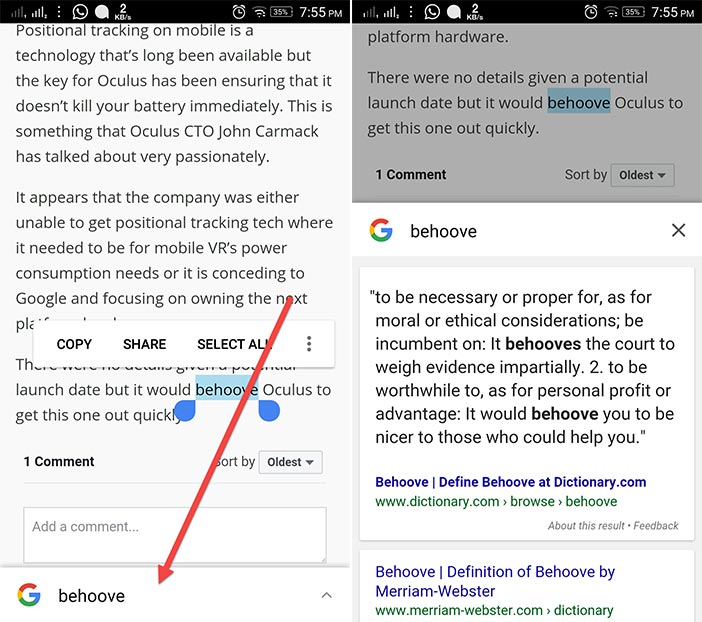This image, captured at 7:55 p.m. from a cell phone, is split into two sections, showcasing a detailed analysis of positional tracking technology for mobile VR and its implications on battery life. The phone's battery is at 35%, and the connection signal is strong.

On the left side of the split screen, a page discusses how Oculus CTO John Carmack has emphasized the challenges of avoiding rapid battery depletion while implementing positional tracking on mobile devices. The text suggests that Oculus may be pivoting its focus either due to the energy consumption issues or in response to competition from Google. A pop-up with options like "Copy," "Share," and "Select All" appears, accompanied by a long red arrow pointing down to the word "behoove."

The right side features a darker gray section with the word "behoove" highlighted in blue. It indicates that no launch date details were provided, but it would be advantageous for Oculus to expedite the release. An explanation of the word "behoove" appears in the right-hand corner, indicating its definition and usage. A Google image icon is also present, enhancing the comprehensiveness of the details provided.